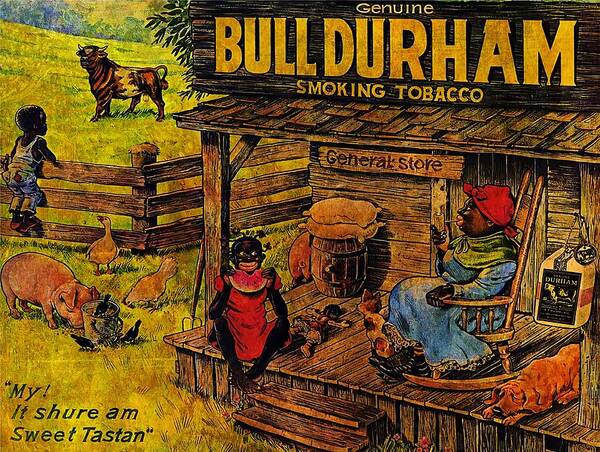The illustration in question is a highly offensive, racist depiction of African-Americans in a rural setting. It portrays a scene outside a dilapidated shack or cabin labeled "Genuine Bull Durham Smoking Tobacco, General Store." A prominently featured black woman, exaggerated with very dark skin, oversized red lips, and a bandana on her head, is seated in a rocking chair, smoking a cigarette. There is a dog resting beside her left and a cat to her right. A young black girl with stereotypically exaggerated features, including large lips and wide eyes, is eating a slice of watermelon nearby. Out in the field, pigs and chickens can be seen, reinforcing the farm setting. Additionally, a black boy with similarly exaggerated dark skin and large lips is perched on a wooden fence, staring at a bull in the pasture. The text at the bottom of this illustration reads, "My, it sure am sweet tastin'," with intentional misspellings to mock African-American vernacular.